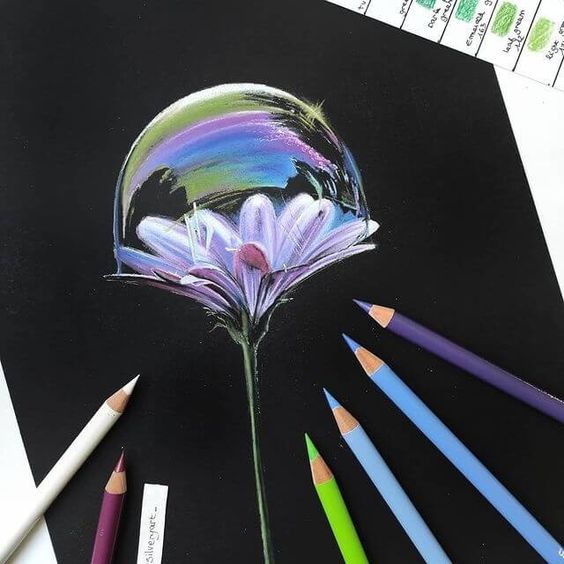The image showcases a highly detailed color pencil drawing on a black paper canvas. Six very sharpened colored pencils—comprising white, two shades of pastel blue, green, purple, and violet—are laid out in a fanned arrangement at the bottom, all pointing toward the focal point of the artwork. The drawing depicts a white-petaled flower with subtle purple and blue accents atop a tall, dark green stem. Atop the flower rests a large, iridescent bubble, rendered with a photorealistic quality, reflecting purples, greens, blues, and yellows to simulate the effect of light shining on it. Additional elements in the image include a piece of paper in the upper right corner with color samples separated by black lines and what appears to be writing in cursive, and another small piece of paper to the lower left labeled "silver jart" or "silver J-A-R-T" with an underscore.